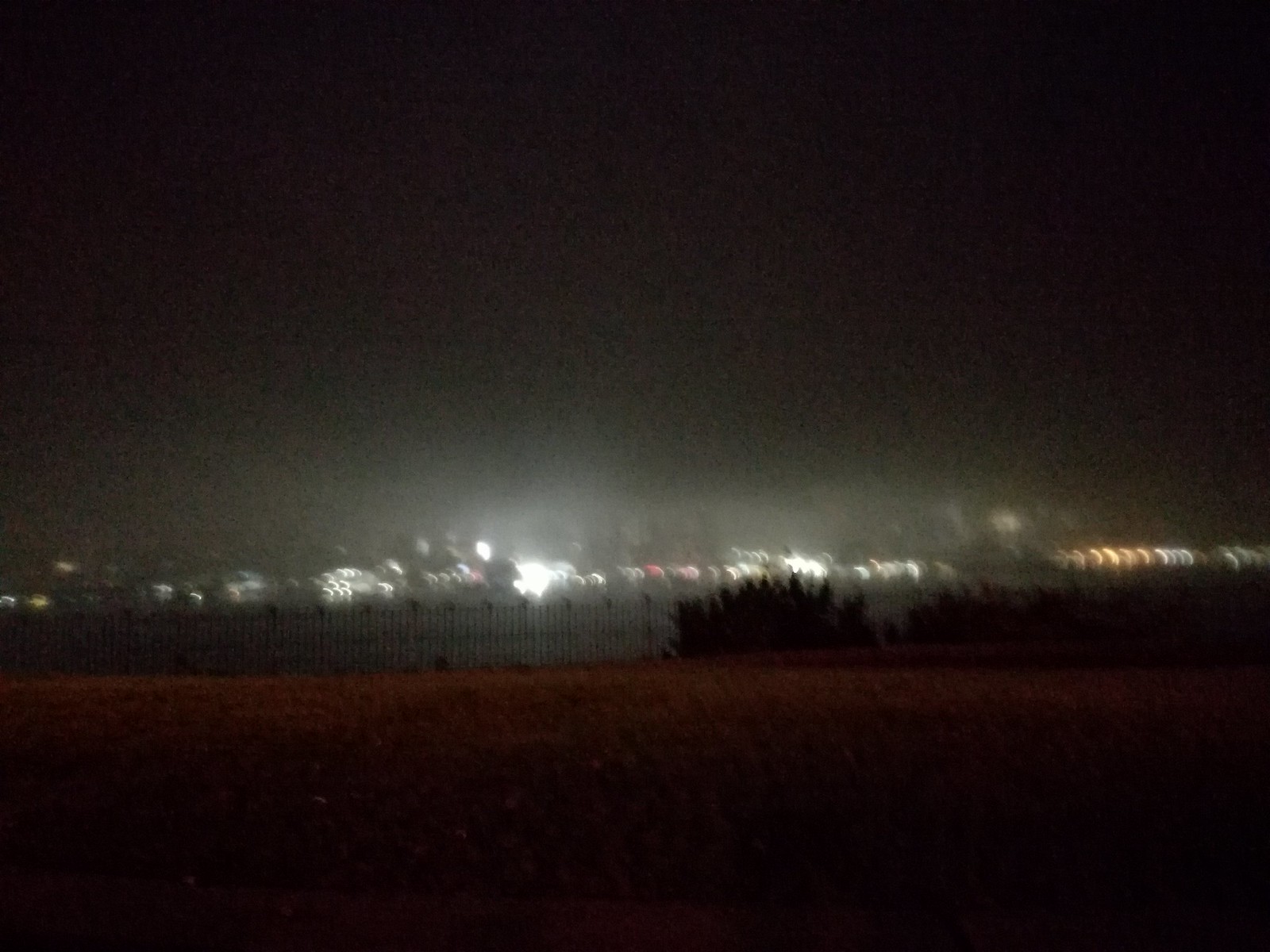This nighttime image, set outdoors, showcases a blurry and somewhat surreal cityscape. The sky is pitch black at the top, gradually transitioning into a grayish hue where the scattered lights begin to appear. The background features a city with glowing buildings, cars, and a myriad of lights emitting white, red, and orange hues, possibly resembling distant city lights blurred into crescent shapes. Near the foreground is a long, large fence characterized by a repetitive pattern of several small poles followed by a thicker one, all shrouded in darkness. Taller dark green bushes rise above the fence, adding to the layered landscape. In the immediate foreground, there is a patch of dark, grassy terrain that fades into black, reflecting the nighttime obscurity. This composite image, with its mixture of natural and urban elements, is rendered in unique blurry detail, potentially suggesting a time-lapse effect, contributing to an almost dreamlike atmosphere.